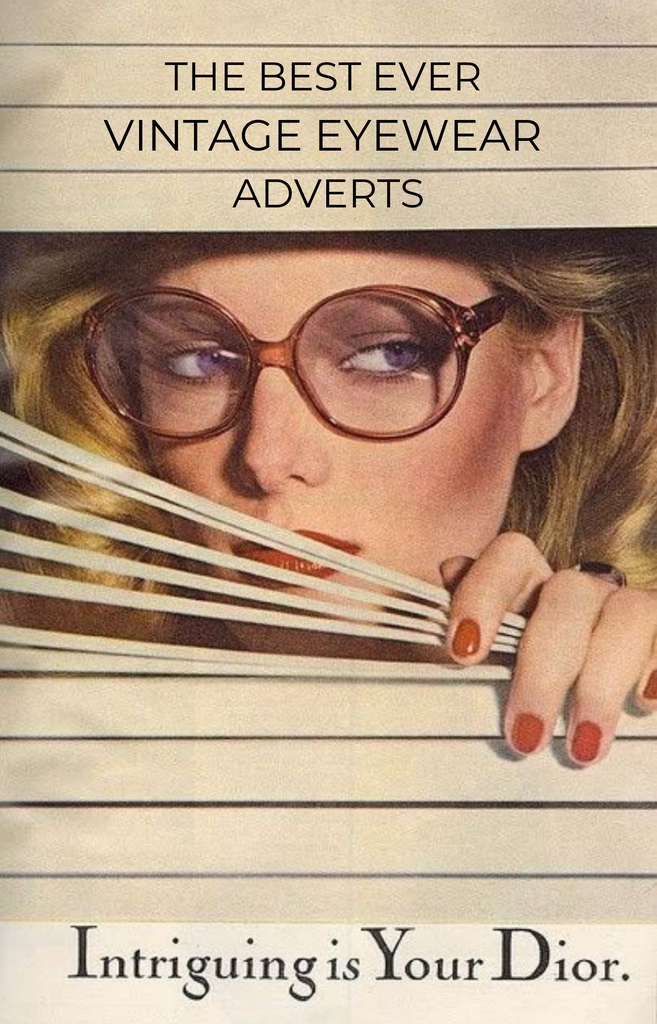The poster is an alluring vintage eyewear advertisement designed to capture attention with its intriguing setup. It features a white Caucasian woman with reddish-blonde hair and striking blue eyes, peering through a set of partially opened white mini blinds. The blinds, closed but pulled down more on the right, frame her face as she looks off to the side. She sports large, thick-rimmed, round eyeglasses with a subtle tint, which accentuates her smoky eye makeup and bright red lipstick. Her visible hand, adorned with bright red nail polish and a ring on her middle finger, grasps the blinds, adding an element of suspense. At the top of the poster, bold black capital letters proclaim, "THE BEST EVER VINTAGE EYEWEAR ADVERTS," while the bottom of the poster reads, "Intriguing is your de Jour," in a more elegant font, with particular emphasis on the I, Y, and D. The overall grayish hue of the mini blinds contrasts with the vibrant details of the woman's appearance, enhancing the vintage charm of the advertisement.